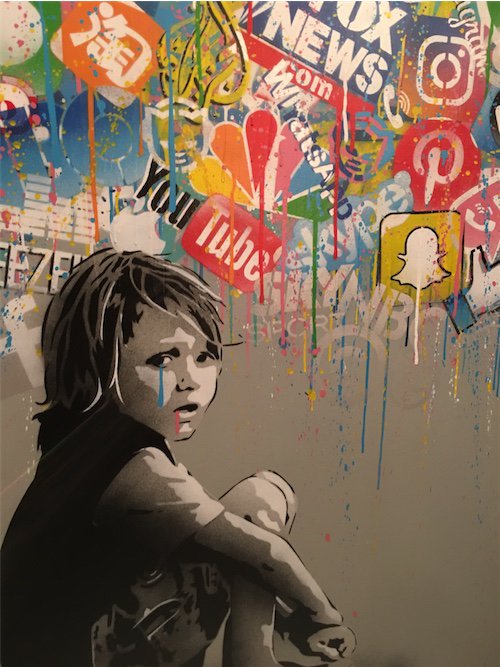This painting portrays a young boy, approximately seven or eight years old, sitting on the ground with his hands clasped around his knees. The child, rendered entirely in grayscale, is gazing directly at the viewer with a distressed and unhappy expression. His hair is neatly parted to the side, and a vivid blue line, resembling a tear, streaks down from his right eye. Additionally, a small red spot is visible at the right corner of his mouth. Surrounding the boy, and contrasting starkly with his monochromatic depiction, are numerous splashes of color in the form of paint splotches—blue, orange, green, red, and yellow—that cascade around him. Above and beside him are an array of brightly colored media and social media logos, including Fox News, foxnews.com (in blue and red text), YouTube, Pinterest, Instagram, Snapchat, and even some icons in Asian scripts. This visual juxtaposition subtly critiques the overwhelming and distressing influence of news and social media on the innocence of childhood.